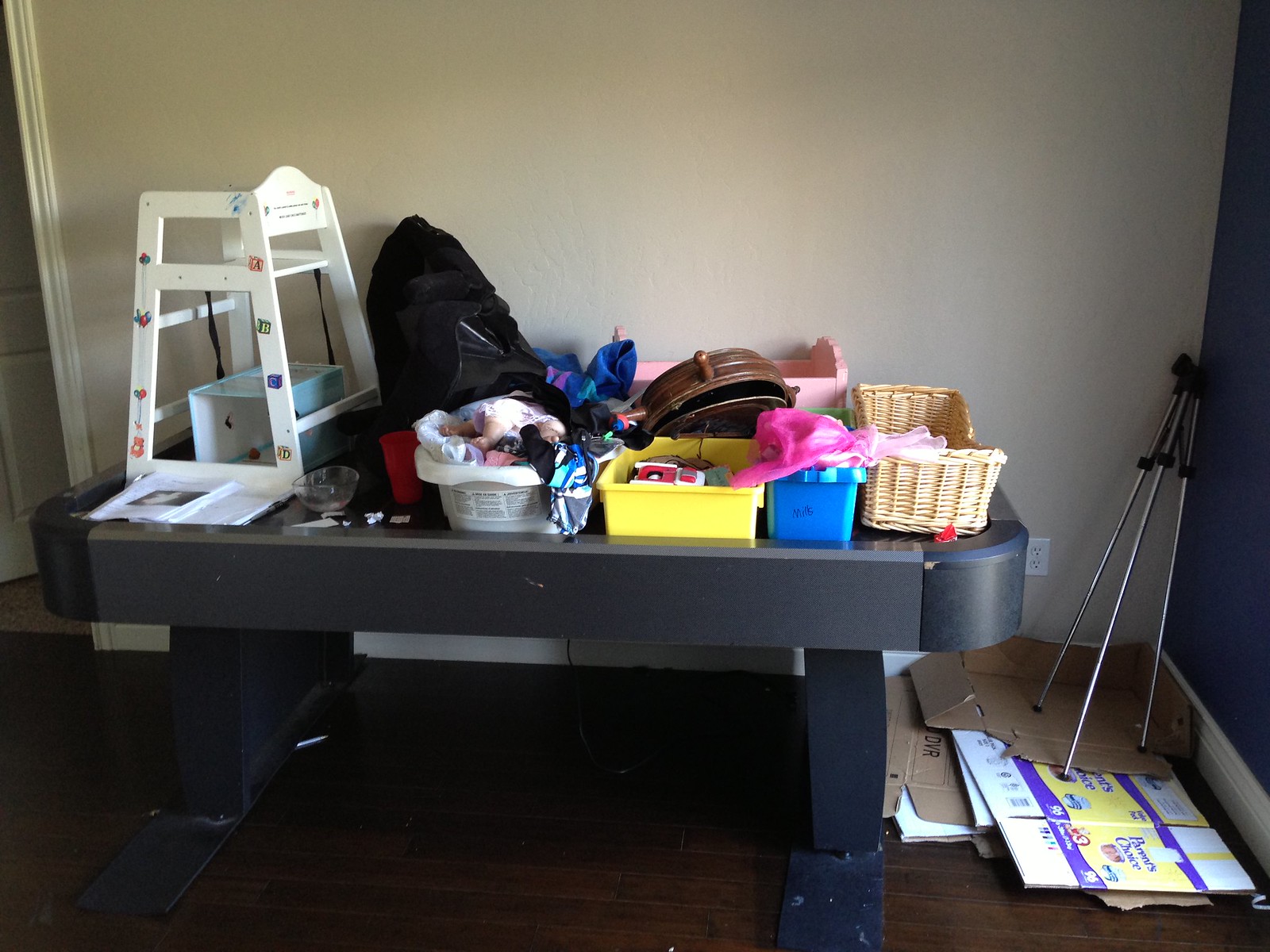In this image, we see a room within someone's house, featuring a black pool table cluttered with various items. The walls are painted in a combination of tan and blue, and adorned with white trim at the bottom. To the left of the pool table, there is an old white high chair decorated with ABC stickers. Beneath the high chair, we observe a white box surrounded by a stack of books. Adjacent to this, a black bag is partially hidden under a pile of clothes that rest in what appears to be an old baby bath. 

Further along, there is a yellow basket overflowing with indeterminate junk and a gold round object of unclear function. Against the back wall sits an old pink baby doll bed. To the right of the yellow basket, a blue plastic container holds what seems to be Barbie doll dresses. At the far right end of the pool table, a wicker basket is placed. On the wooden floor beneath the table lies some broken-down cardboard boxes, alongside what looks like a telescope holder or possibly a metal camera tripod in the room’s corner. The room's arrangement suggests a chaotic mix of items, indicative of an area used for storage.